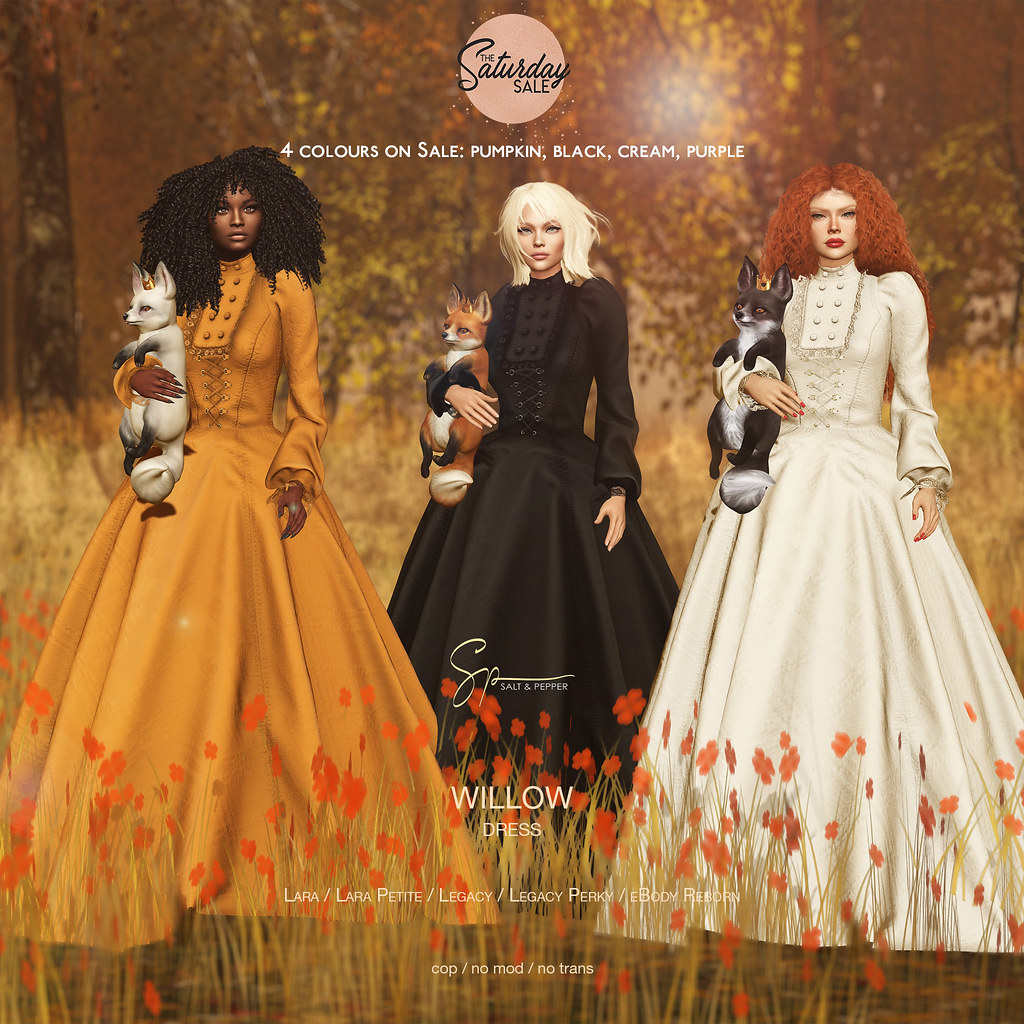This computer-generated, horizontally aligned rectangular advertisement for a sale features a richly detailed, fine art-style scene with a distinct European aesthetic. Set against a forest backdrop awash with autumn hues of yellow, green, and orange, the image fades into a tan-colored field. A prominent circle at the top center contains the text "The Saturday Sale" in cursive.

In the foreground, three computer-generated women, resembling characters from a video game, each hold an animal in their right hand. The African American woman on the left wears a long orange dress and holds a small white dog; she has very curly, long afro hair. The middle figure is a blonde Caucasian woman in a black dress, holding a fox. The rightmost figure, another Caucasian woman with thick red hair styled in a bob, dons a white dress and holds a black and white dog. All of the dresses are long-sleeved with laced-up designs in the center, giving them a Victorian flair.

Below the circular banner, in white text, the advertisement highlights the sale with the message "Four colors on sale: Pumpkin, Black, Cream, and Purple." Near the bottom, layered over the orange flowers decorating the lower part of the image, the text "Willow Dress" stands in bold white letters, followed by a list of compatible body types: "Lara, Lara Petite, Legacy, Legacy Perky, and eBody Reborn." The restrictions "Cop, Nomad, No Trans" appear at the very bottom of the ad.